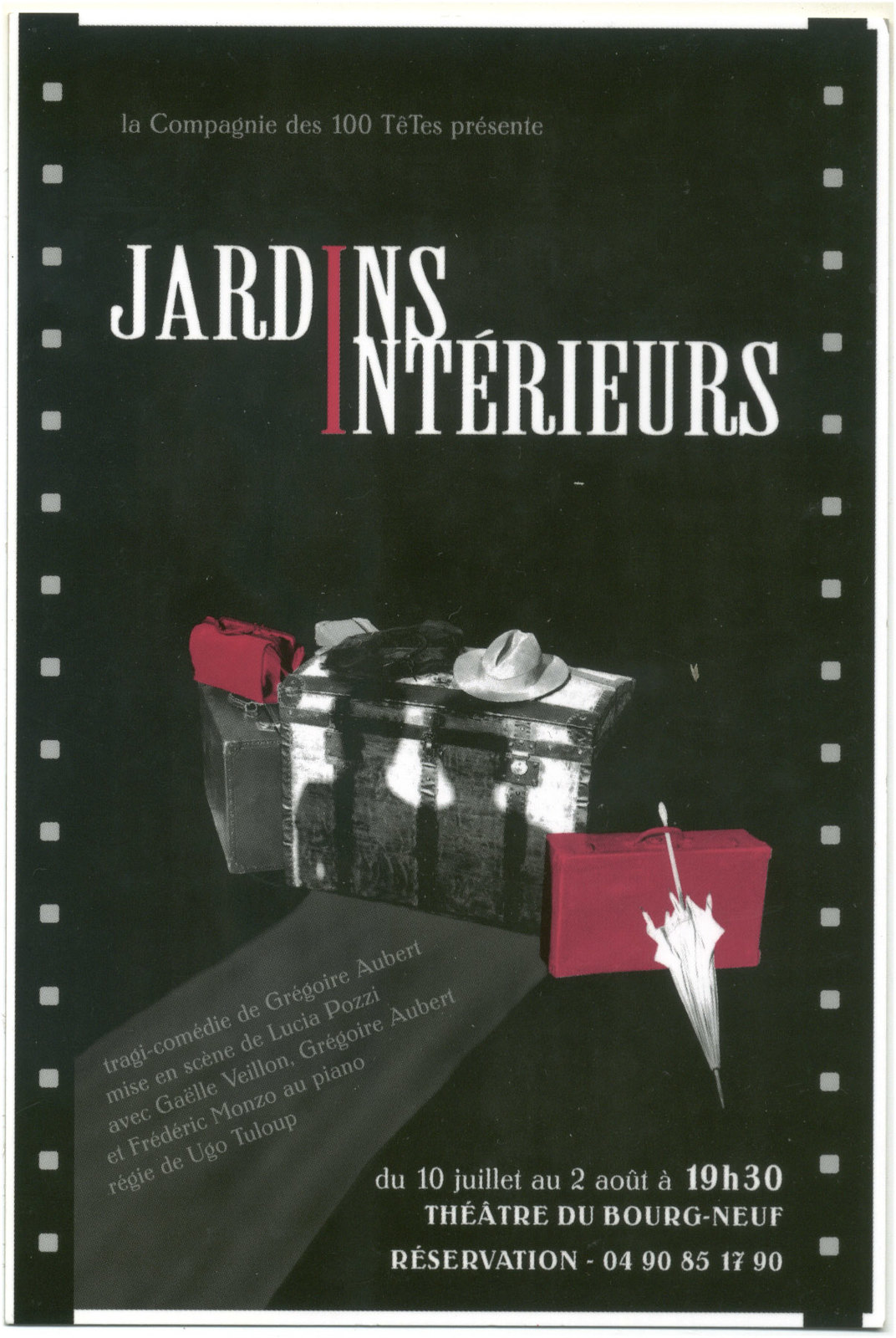The image is a detailed French film poster with a design resembling a strip of film, indicated by vertical lines of gray squares on the left and right sides representing film holes. The background is predominantly black. At the top left, in light gray text, it reads "La Compagnie des Cent Tétés Présente." Below this, the film's title "Jardins Intérieurs" is displayed in white, with a unique feature where the letter 'I' in "Jardin" and the start of "Intérieur" form one large red 'I’. Surrounding the title are various monochrome objects, notably several suitcases of varying sizes, with a couple of red suitcases and a white umbrella threaded through a suitcase handle. A gray hat is also placed on one of the suitcases. Near the bottom, additional information is presented in gray and white text, including details about the film's showing time and location: "Dutte Juliette et Toit, 19H30, Théâtre de Bourgneuve, Réservation, 49085, 1790." The poster's overall aesthetic is primarily black and white with striking red accents.